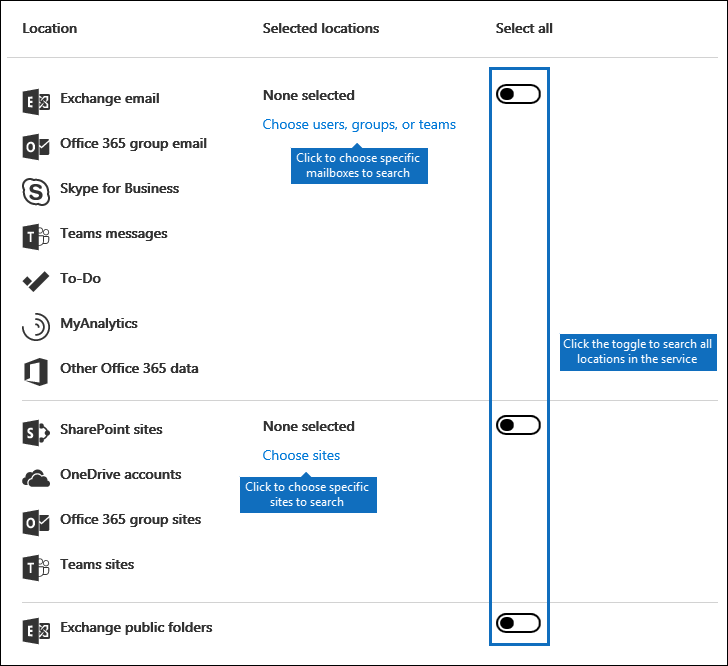This screenshot showcases an Outlook settings page, specifically focusing on location-related configuration options. In the top left corner, the section is labeled "Location," listing numerous Outlook services such as Exchange Email, Office 365 Group Email, Skype for Business, Teams Messages, To Do, My Analytics, Other Office 365 Data, SharePoint Sites, OneDrive Accounts, Office 365 Group Sites, Teams Sites, and Exchange Public Folders.

Beneath this, the interface shows two categories: "Selected Locations" and "Non-selected." Users are prompted to "Choose Users, Groups, or Teams" and can specifically select mailboxes to search. Another segment invites users to "Choose Sites" and pick specific sites to include in their search parameters.

In an additional section titled "Select All," a noticeably highlighted vertical rectangular box contains three buttons, all currently set to "off." Accompanying instructions encourage users to "click the toggle to search all locations in the service."

The page appears to be part of an instructional manual or aid, designed to help users navigate and utilize various Outlook services effectively. This is evidenced by the presence of instructional boxes adjacent to multiple options, providing guidance on their functionality and usage.